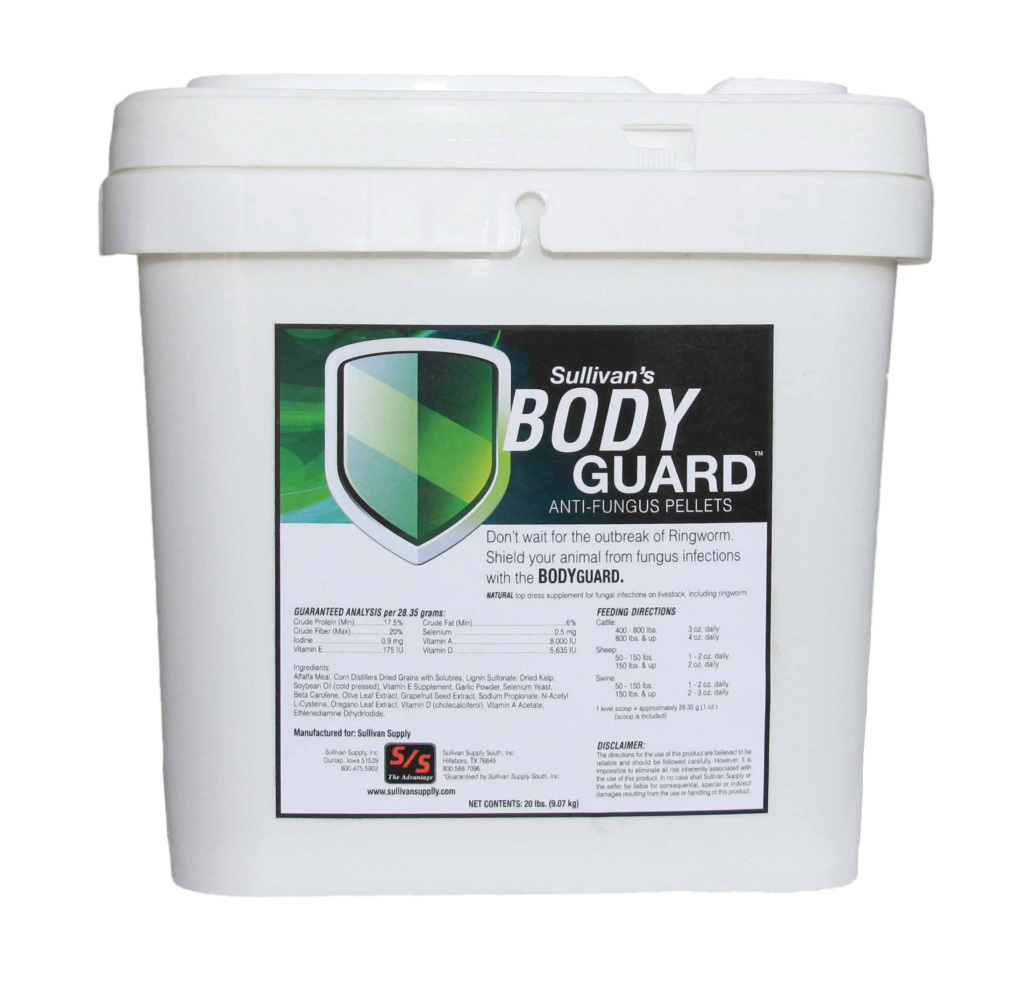This image depicts a nearly square, white product box with a secure lid. At the center of the box is a square label featuring detailed information. Prominently displayed in bold letters at the top right of the label is the product name: "Sullivan's Bodyguard Anti-Fungus Pellets." On the top left, there is a green logo. Below the product name, the label includes a message urging, "Don’t wait for the outbreak of ringworm. Shield your animal from fungus infections with the Bodyguard." The label also provides detailed descriptions of the pellets and instructions for feeding different animals, including cattle, sheep, and swine. The outline of a dark green shield with silver accents adds a distinctive visual element to the label. A manufacturing logo is located at the bottom left of the label.